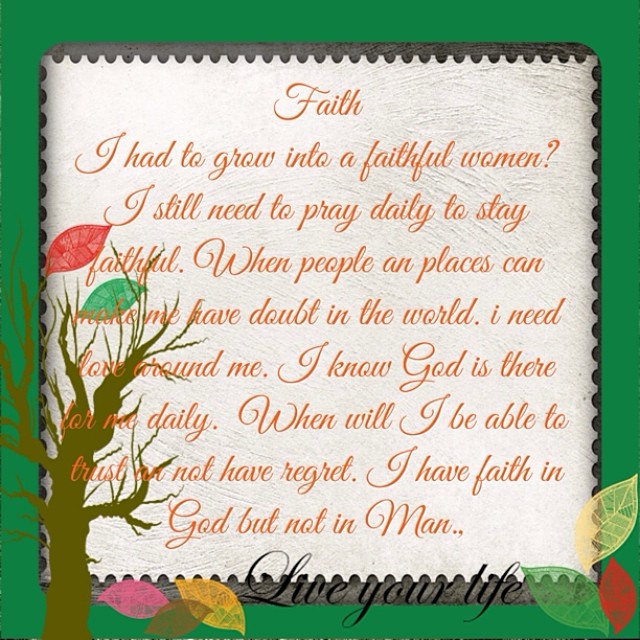The image resembles a decorated plaque or the cover of a greeting card with a white background and a green border. In the lower left corner, there is a clip-art style tree adorned with leaves in various colors—red, green, pink, brown, orange, and yellow. Orange cursive text in the center reads: "Faith. I had to grow into a faithful woman. I still need to pray daily to stay faithful. When people in places can make me have doubt in the world, I need love around me. I know God is there for me daily. When will I be able to trust and not have regret? I have faith in God but not in man."